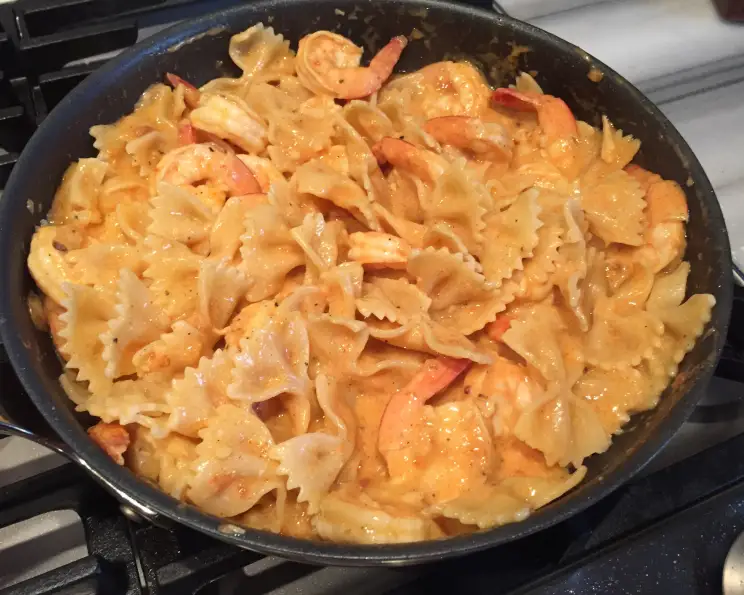The photograph captures an indoor scene featuring a black cast iron skillet positioned on the edge of a silver and black stove, likely with black grates and a gray top surface. The skillet is filled with bow tie (farfalle) pasta, which is tan and ridged at the ends, coated in a shiny, cheesy sauce. The pasta is mixed with non-breaded, cooked shrimp, still with their tails on, and sprinkled with black pepper and possibly some salt. The creamy sauce has a subtle tomato tint, adding to the rich texture and color of the dish. The overall background hints at a modern kitchen setup, focusing the viewer's attention on the delectable contents of the skillet.